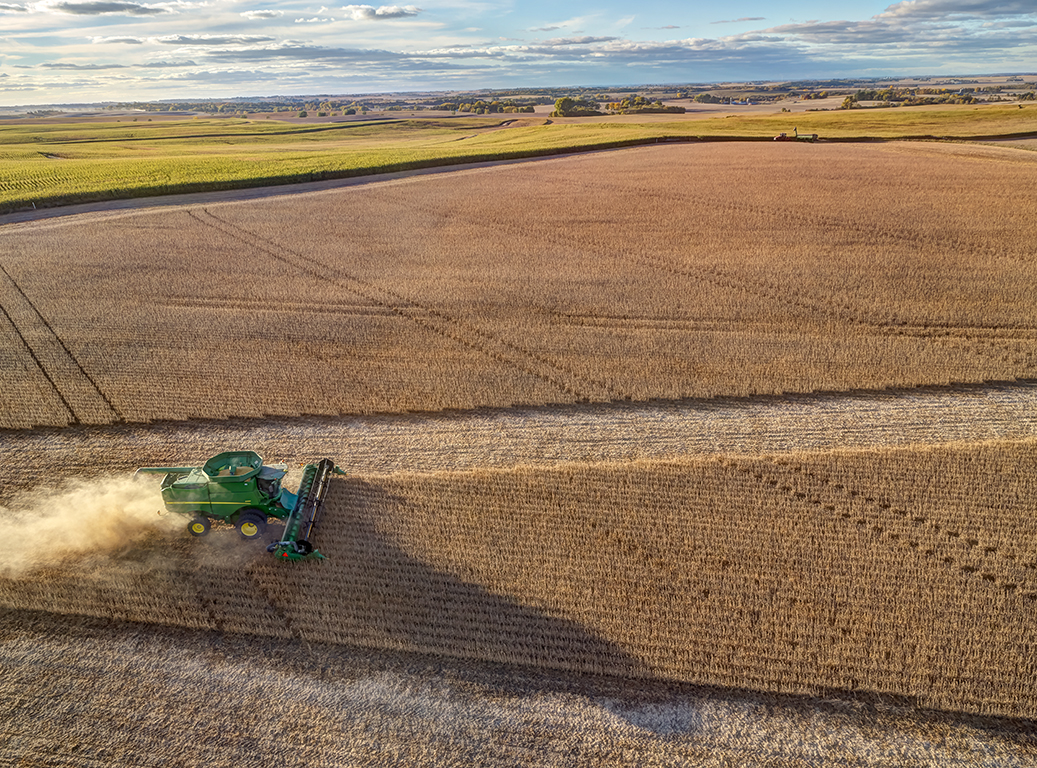This image captures an expansive aerial view of a vast field primarily filled with golden-brown crops, likely wheat. Dominating the scene is a green tractor with yellow rims and a wide mouth attachment, actively harvesting the crop. The tractor is positioned towards the left side of the frame, moving from left to right, evidenced by the clear zigzag tracks it leaves behind in the lower half of the image, where the grain has already been harvested. The field extends outwards, revealing a patchwork of mowed and standing grain. Surrounding the main field are sections of greener grass and additional farmland, dotted with trees and faintly visible buildings in the distance. The sky overhead is a mix of blue with scattered clouds, suggesting either a recent or upcoming storm, with the sun faintly peeking through on the left. This detailed landscape showcases the agricultural activity and the serene yet industrious rural environment.